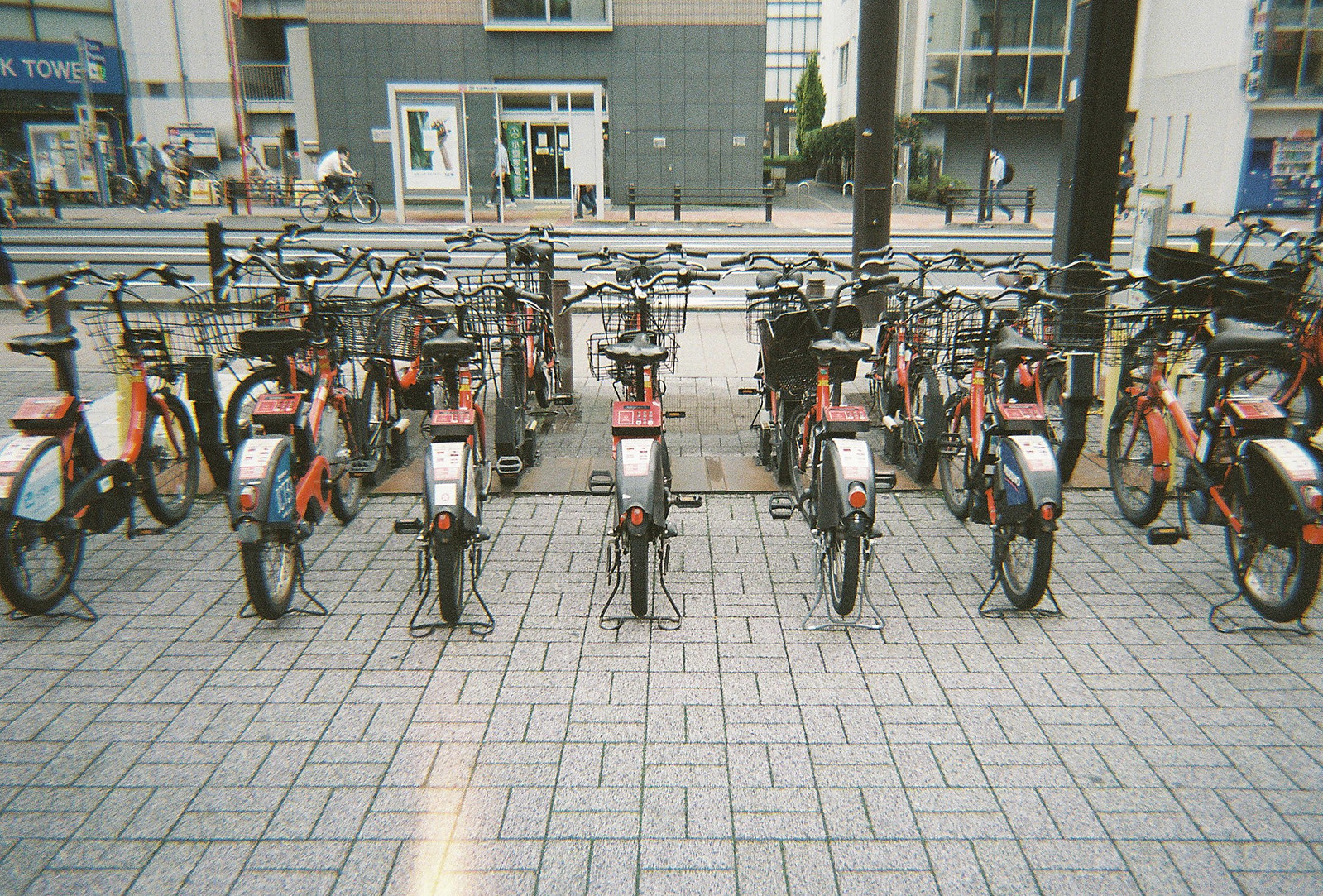The image captures a bustling city scene, potentially in Japan, featuring rows of red bicycles with black seats and tires, neatly parked on a gray brick sidewalk. These bikes appear to be available for public rental, indicated by their number pads and small text boxes, likely for payment. Each bike is equipped with a wire basket at the front. In the foreground, the bicycles are arranged in parallel lines against a metallic rack. Beyond the bikes, there’s a city street lined with various buildings, one notably displaying a partially obscured "Tower" sign in white letters on a blue background. The busy urban backdrop includes pedestrians, some of whom are wearing masks, a bus stop, and a vending machine. Visible among the crowd is a person biking wearing a white shirt and people leisurely walking. The overall ambiance reflects a typical vibrant downtown atmosphere with a mix of modern infrastructure and everyday city life.